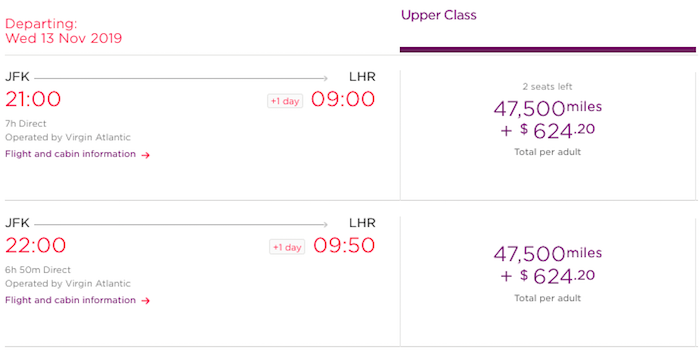***Descriptive Caption:***

This webpage image is from a travel booking site, specifically for flight reservations. The main header indicates a departure on Wednesday, November 13th, 2019. 

In the upper left corner, highlighted in red, the text says "Departing." Below this, it details a flight from JFK Airport at 2100 hours (9:00 PM), with a notation "+1 day, 9 hours," indicating a subsequent arrival at LHR Airport after a total travel time of 7 hours for a direct flight. The flight is operated by Virgin Atlantic.

Beneath this, another flight option is listed:
- Departure from JFK at 2200 hours (10:00 PM).
- Noted as "+1 day," with an arrival at LHR at 0950 hours (9:50 AM).
- This flight duration is 6 hours and 50 minutes, also a direct flight, operated by Virgin Atlantic.

Both flight options include a section labeled "Flight and Cabin Information" in purple, accompanied by a red arrow.

On the right side of the image, details regarding Upper Class seating are provided. The Upper Class label is displayed in a purple bar, with a note highlighting only two seats left. Each flight option costs 47,500 miles plus an additional $624.20 per adult. Thus, both flights share the same pricing scheme.